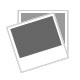This image is a detailed illustration of a particular font set, showcasing both letters and numbers. The design includes uppercase and lowercase versions of 'A' and 'B', followed by the numbers '1', '2', '3', and '4'. These characters are computer-generated and displayed in a black and white color scheme, with a textured, chalk-like appearance featuring diagonal white lines inside the characters. Each letter and number is outlined with a black border. The sequence of 'A', 'a', 'B', 'b', '1', '2', '3', '4' repeats three times in vertical columns from the top to the bottom of the image, totaling 24 characters. The background appears to be white, and the style is reminiscent of cutouts from a newspaper or magazine, suggesting it might serve as a sample for potential text design or a template for alphanumeric decals.